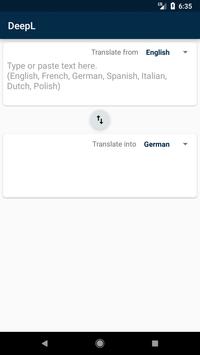The image features a screenshot of a mobile phone displaying the DeepL translation website. In the top right corner, the time indicates 6:35, accompanied by nearly empty battery and two-bar phone signal strength icons, both colored in white. To the left, the word "DeepL" is prominently displayed in white, with a dark blue background, and both the 'D' and 'L' in uppercase.

Below the header, a box contains the text "Translate from English," where "English" is in dark black and "translate from" in light gray, with a drop-down arrow beside it. On the middle left of the box, instructions to "Type or paste text here" are listed, followed by a series of languages: English, French, German, Spanish, Italian, Dutch, and Polish. Further down, a circular icon with an up-and-down arrow is present, indicating translation direction. Below it, another box reads "Translate into German."